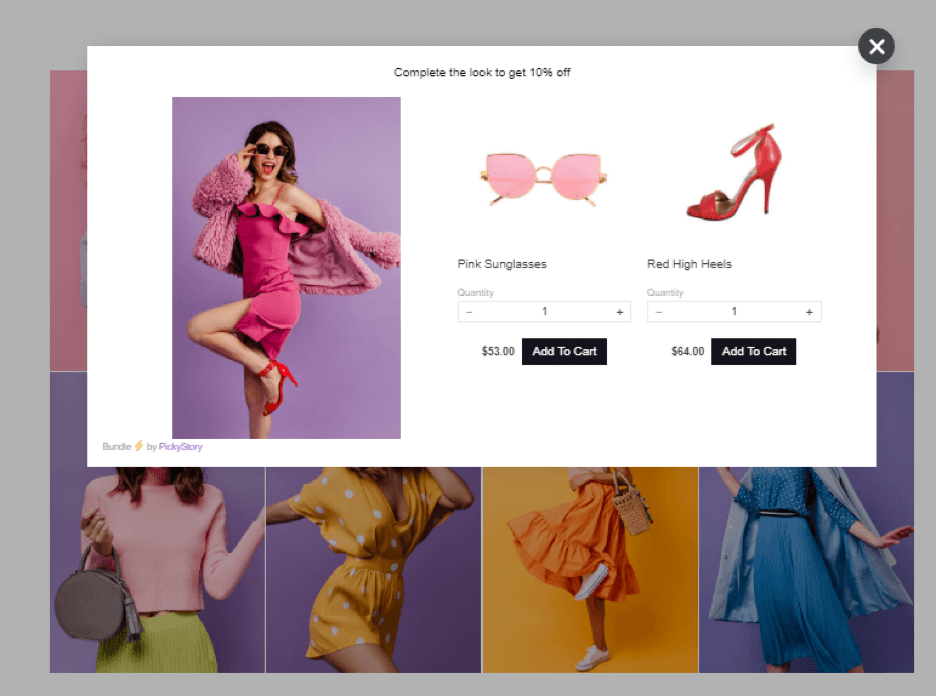This is a screenshot from a clothing website, featuring a centralized long rectangular white box. Inside this box, on the left side, there is an image of a woman posing in front of a purple background. She is dressed in a bright pink short dress, complemented by a pink fluffy jacket and red high heels. She wears pink sunglasses and has glasses on while playfully sticking her tongue out.

To the right of her image, the items she is wearing are showcased individually. The first item is a pair of pink sunglasses, detailed with black text reading "Pink Sunglasses." Next to the sunglasses, there is a single red high heel, annotated with black text that says "Red High Heels." Below each description, there is a quantity box, and beneath that, a black square button with white text that reads "Add to Cart."

Behind this central box, several other images of women in various outfits are displayed, creating a vibrant fashion collage. In the bottom left, one woman wears a long-sleeve short pink shirt paired with a lime-green skirt, holding a light gray bag in her right hand. Moving to the right, the next woman is dressed in a short yellow dress adorned with white polka dots. Further right, another woman is seen in an orange dress, carrying a basket-like purse. Finally, in the bottom right corner, a woman wears a longer blue dress, accompanied by a coordinated long blue jacket draped behind her.